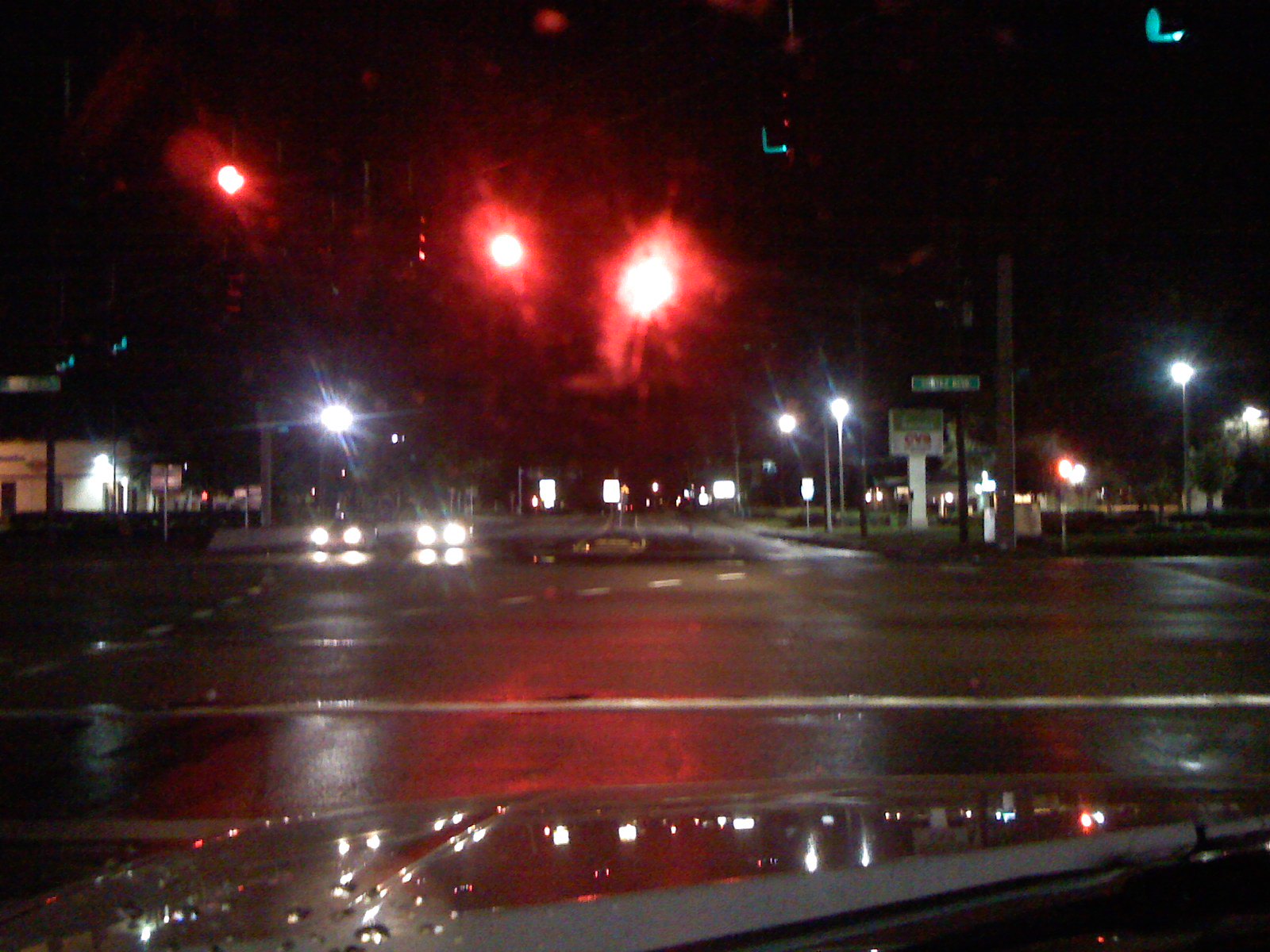The color photograph, taken from the first-person perspective of a driver, showcases a nighttime or early morning scene at an intersection. The sky is pitch black, indicating the time, and the wet ground suggests it has recently rained, with water droplets visible on the windshield and hood of the dark vehicle. Visible through the front window, three glaring red traffic lights are suspended above, indicating the vehicle is stopped. The intersection features multiple lit street lamps, both illuminating the road and reflecting off the damp pavement. On the left, there's a building and a white billboard, while green and white road signs can be seen on the right. Ahead, two cars with their headlights on are positioned in the opposite lanes, reinforcing the wet road conditions. The overall scene is detailed by the reflections and light glares, providing a vivid snapshot of a quiet, wet night at a city intersection.